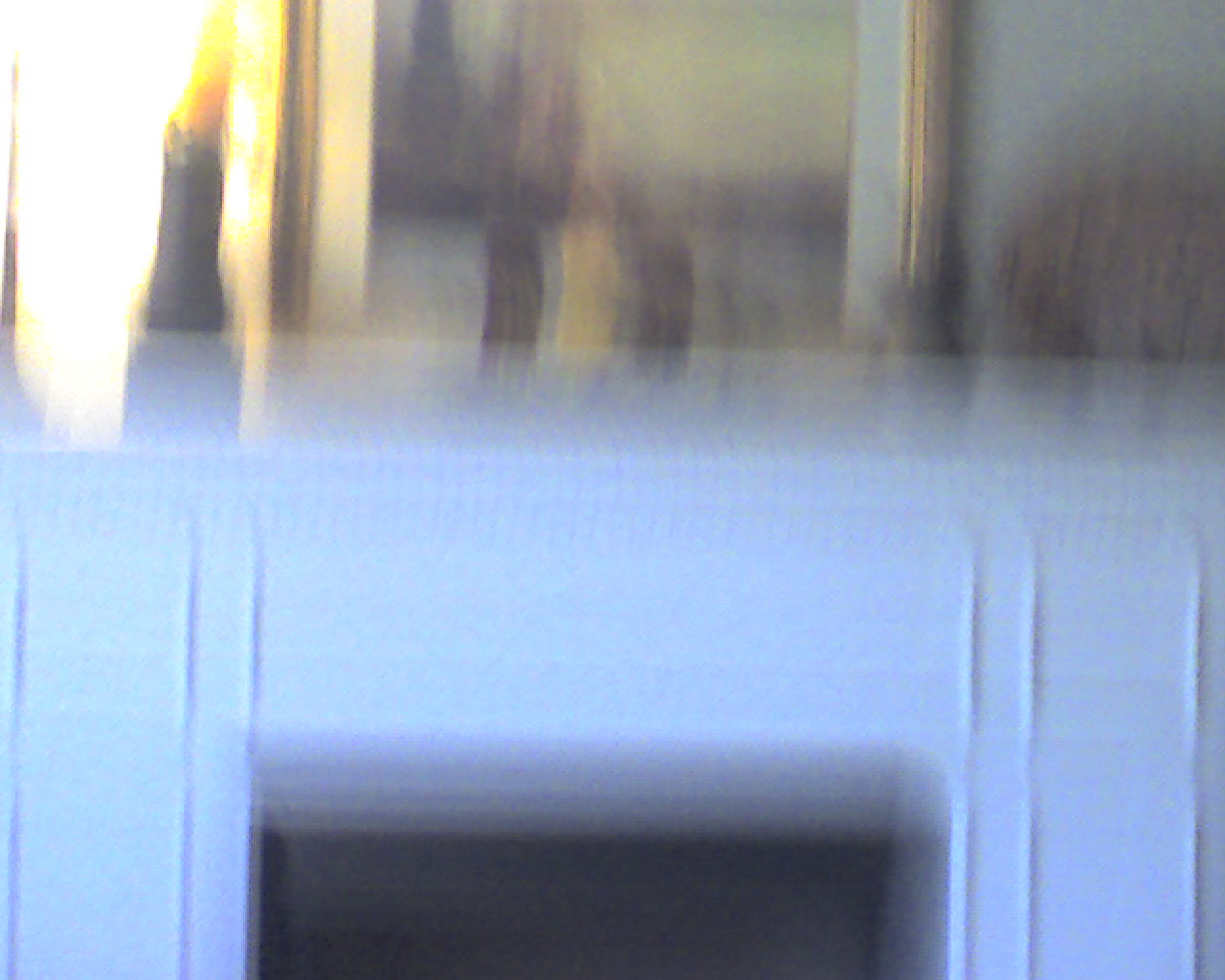This is a very blurry color photograph of a white fireplace taken inside someone's house. The grainy, out-of-focus image reveals a significant quality issue, possibly due to camera movement or a dirty lens. The white fireplace has a distinct black rectangular opening at its center. There are two vertical lines on either side and two horizontal lines above the opening, adding subtle detail. The fireplace is flanked by a white arch-like mantle. On the mantle rests a gold-framed painting, although its contents are indistinguishable due to the photograph's poor quality. Hints of other objects, such as what might be a flower or a candle, appear next to the painting, but they are too blurry to be identified clearly. The overall scene lacks any people, animals, plants, or mechanical objects.